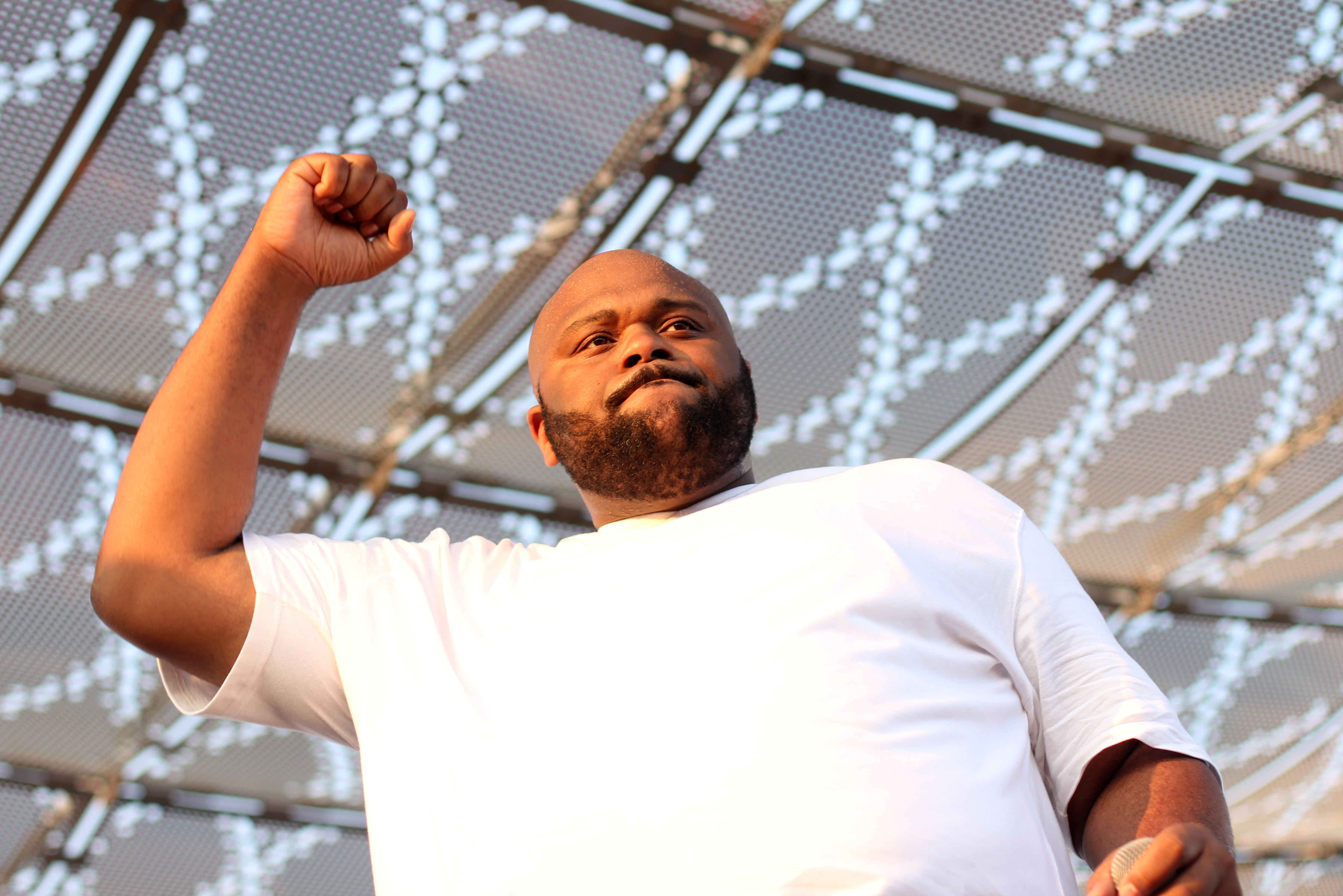The image depicts an African-American man who appears to be performing at an outdoor event, possibly a concert. He is bald and has a distinct, full black beard and mustache. His right arm is raised with a closed fist, and his left hand is gripping a microphone, identifiable by its grayish ball with dots. He is dressed in a white short-sleeved shirt. The photograph is taken from a low angle, suggesting that the man is elevated, possibly on a stage, and the viewer is part of the audience. Above him, a metallic grid structure forms a canopy with netting sheets, featuring a diamond and X-patterned design. The scene is lit by natural sunlight, casting shadows that indicate it is daytime.